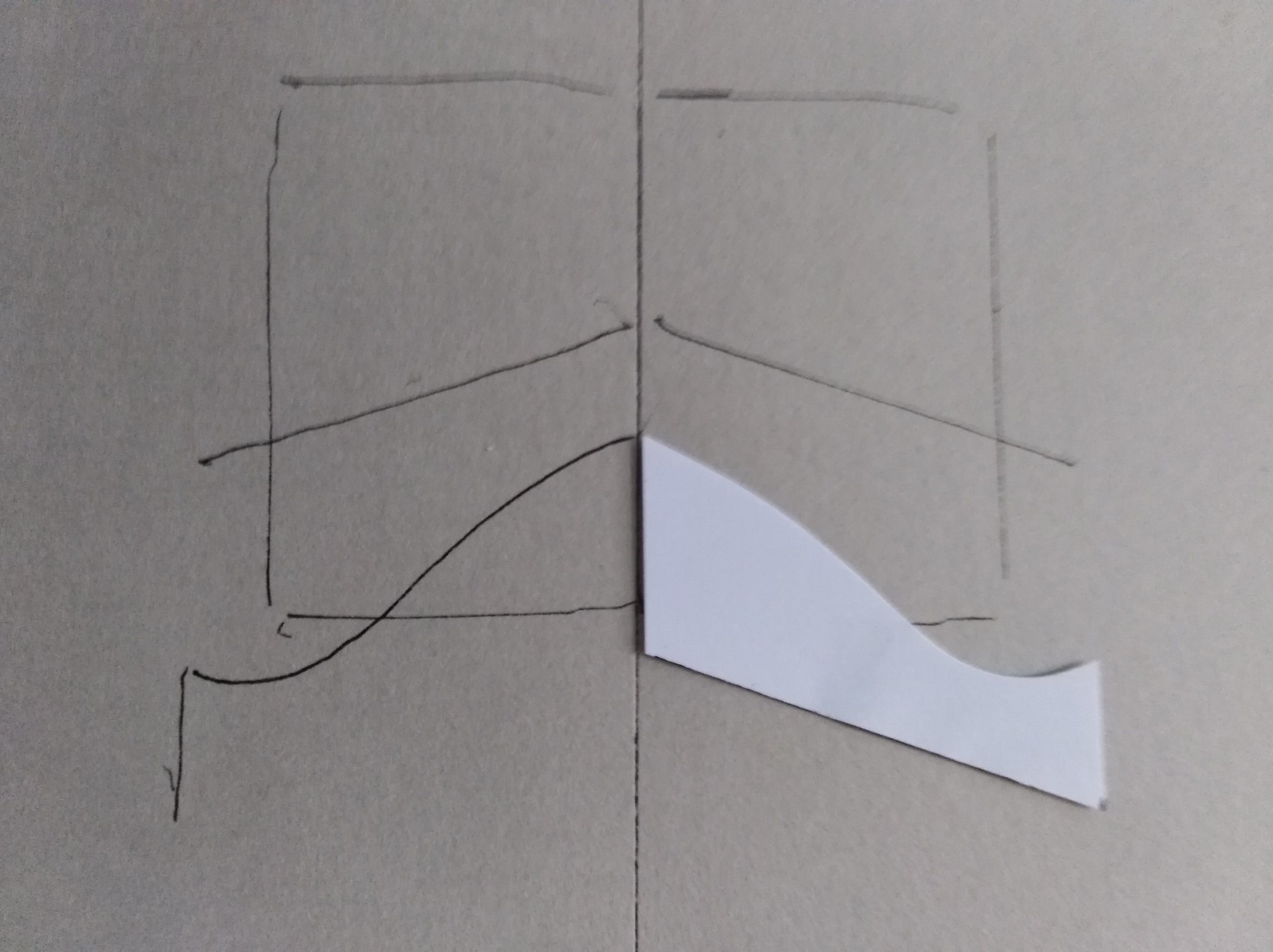The photograph captures a single piece of gray cardboard, similar in texture and appearance to the stiff back cover of a legal pad. A prominent vertical line runs from the top to the bottom of this cardboard, dividing it into two equal halves. On each half of the cardboard, a diagonal line extends from the central vertical line towards the outer edges, creating a shape that resembles a shallow roof.

Each half of the cardboard has a separate, slightly curved template positioned on it. The white template, which appears to be made of either cardboard or plastic, is characterized by a curved top edge, with straight edges on the bottom and the left side. The template on the left side has already been traced, evidenced by a defined outline along the lines. The right side is in the process of being traced, starting from the vertical line that splits the cardboard.

The arrangement and tracing of these templates, when completed, will form a design similar to a headboard, with the symmetrical halves meeting at the central vertical line, creating a cohesive and detailed representation.